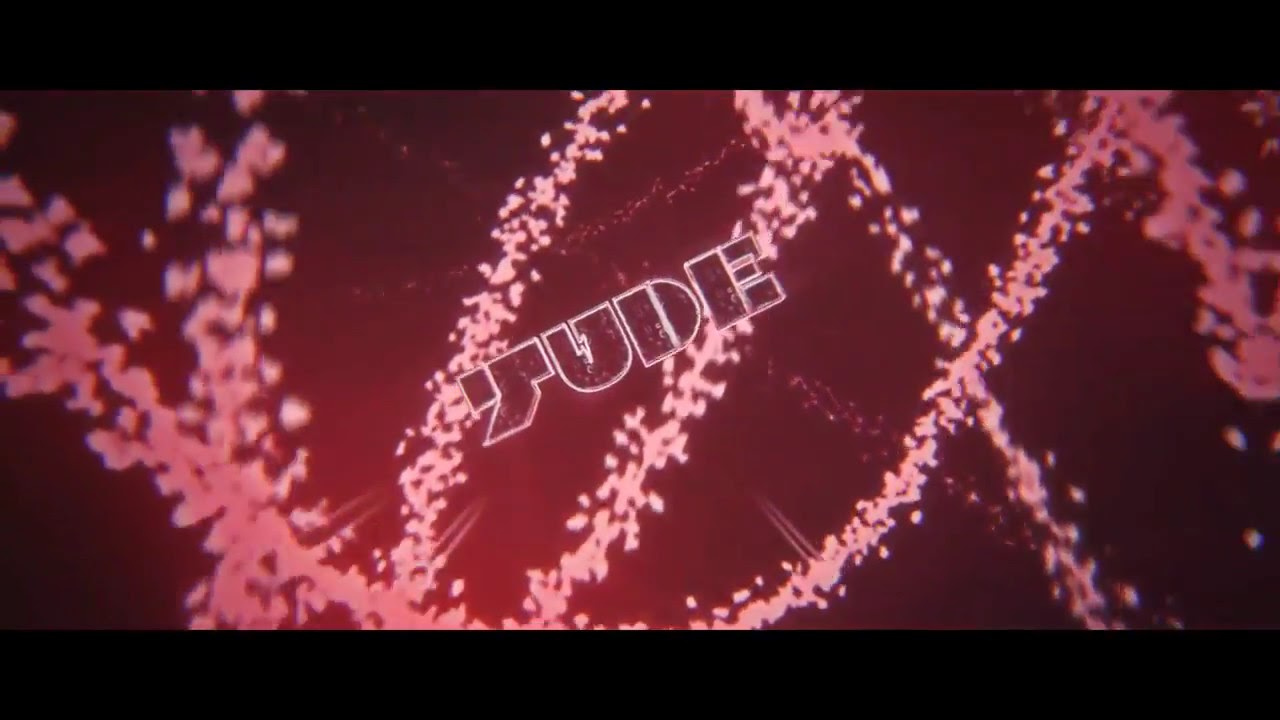The image is a digital artwork or page with a dark, maroonish, and reddish-pink background. It has black horizontal borders at the top and bottom, forming a rectangular letterbox shape. Centered in the middle of the image, there are bold, capitalized block letters spelling "JUDE" in red with a white outline. The initial letter, which is a stylized J, is slightly cut off on the left side, making it resemble a T. A unique lightning bolt detail adorns the top of the U. The background features scattered, streaking pink elements that resemble flower petals or string lights, arranged in various crisscrossing and curvy patterns, contributing to a dynamic and somewhat blurred visual effect.